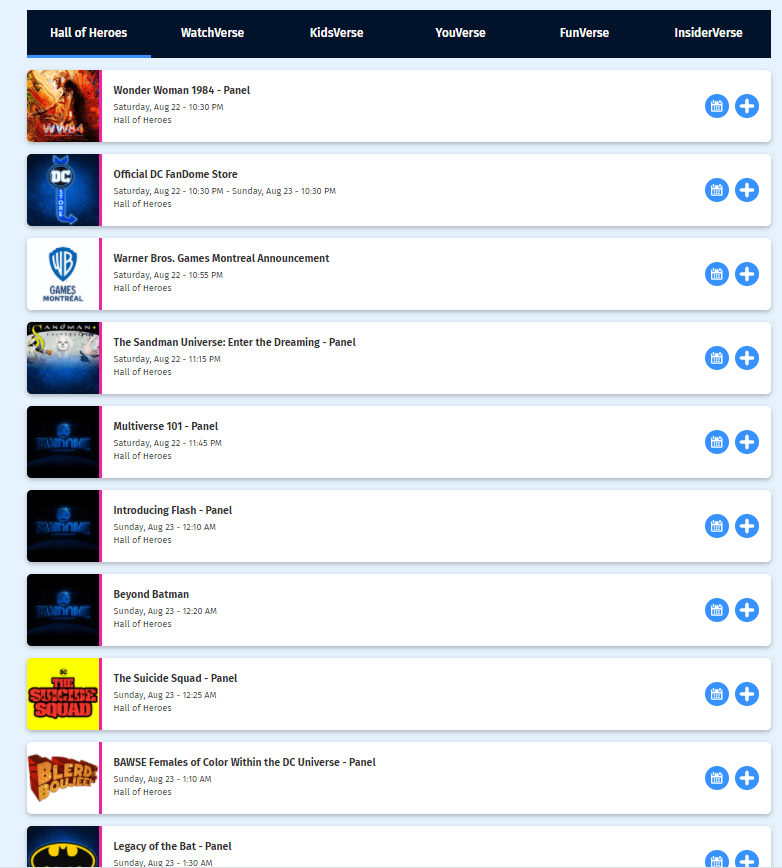This document serves as a schedule for sci-fi enthusiasts, detailing various events and panels under the DC Fandome categories: Hall of Heroes, Watchverse, Kidsverse, U-verse, Funverse, and Insiderverse. Here are the noteworthy events listed with their respective times:

- **Wonder Woman 1984 Panel**: Saturday, August 22nd at 10:30 PM in the Hall of Heroes.
- **Official DC Fandome Store**: Sunday, August 23rd at 10:30 PM.
- **Warner Brothers Games Montreal Announcement**: Saturday, August 22nd at either 10:35 PM or 10:55 PM.
- **The Sandman Universe - Enter the Dreaming Panel**: Saturday, August 22nd at 11:15 PM.
- **Multiverse 101 Panel**: Saturday, August 22nd at 11:45 PM.
- **Introducing Flash Panel**: Sunday, August 23rd at 10:12 AM.
- **Beyond Batman**: Sunday, August 23rd at 12:20 AM in the Hall of Heroes.
- **Suicide Squad Panel**: Sunday, August 23rd at 2:25 AM.
- **Females of Color Within the DC Universe Panel**: Sunday, August 23rd at 1:10 AM.
- **Legacy of the Bat Panel**: Sunday, August 23rd at 1:30 AM.

This schedule helps fans track their favorite events and panels.